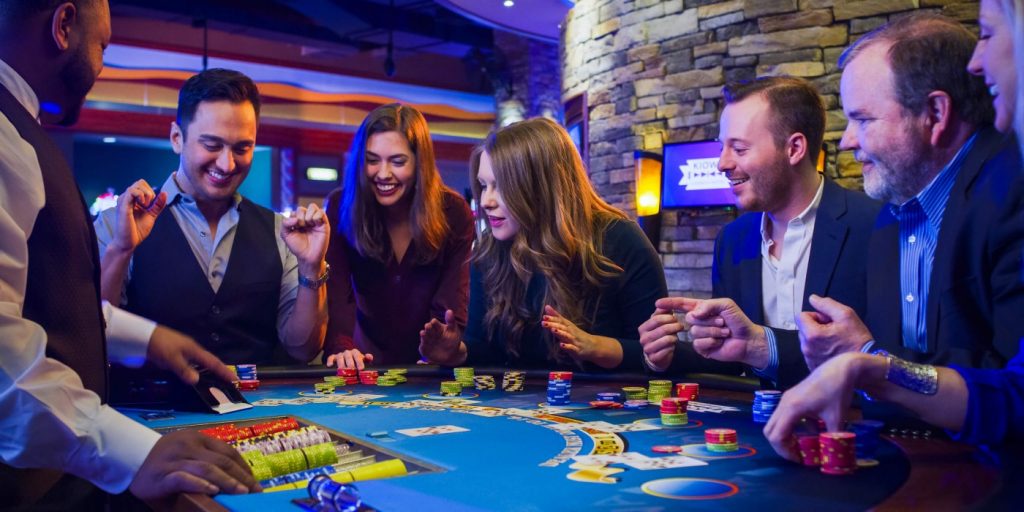The indoor image depicts a lively casino scene at nighttime, illuminated by the room's lights. Central to the scene is a blue blackjack table brimming with colorful chips and playing cards. Positioned on the left is the dealer, a Black man dressed in a white shirt and black vest, standing behind the table's chip compartment. Surrounding the table, there are five patrons: starting from the left, a cheerful man with his hands raised, exuding the excitement of a recent win, followed by two women with brown hair, another man, and a final woman partially visible in the upper right corner of the image.

In the backdrop, a stone fireplace and a tan and gray brick wall add a rustic touch to the otherwise modern setting, adorned with a neon sign and a TV monitor. The group's attention is collectively focused on the jubilant man on the left, sharing in his moment of triumph with beaming smiles. The scene captures the thrill and camaraderie typical of a casino atmosphere.